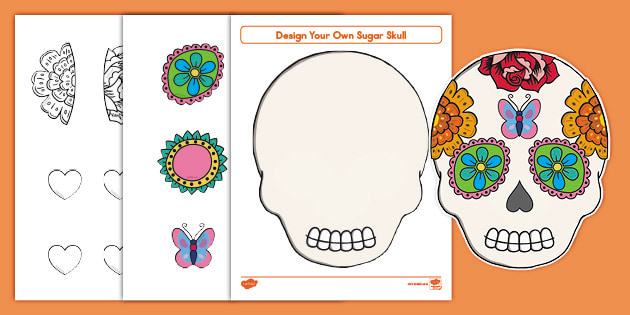The image is a digital graphic from a website, featuring a child's craft project with a vibrant orange background. On this backdrop, three overlapping sheets of paper are displayed, each casting a drop shadow. The top sheet prominently showcases a skeleton face with an emphasis on the teeth, accompanied by the text "Design Your Own Sugar Skull." This design resembles a Day of the Dead sugar skull, depicted in a step-by-step format. Some designs are pre-colored, while others are black and white, intended for personal coloring. Additional sheets offer various stickers, including flowers, butterflies, and hearts, for decorating the skull. The final completed sugar skull, featuring colors like green, blue, and orange, can be seen on the right-hand side of the image. The nose of the skull notably resembles an upside-down heart.